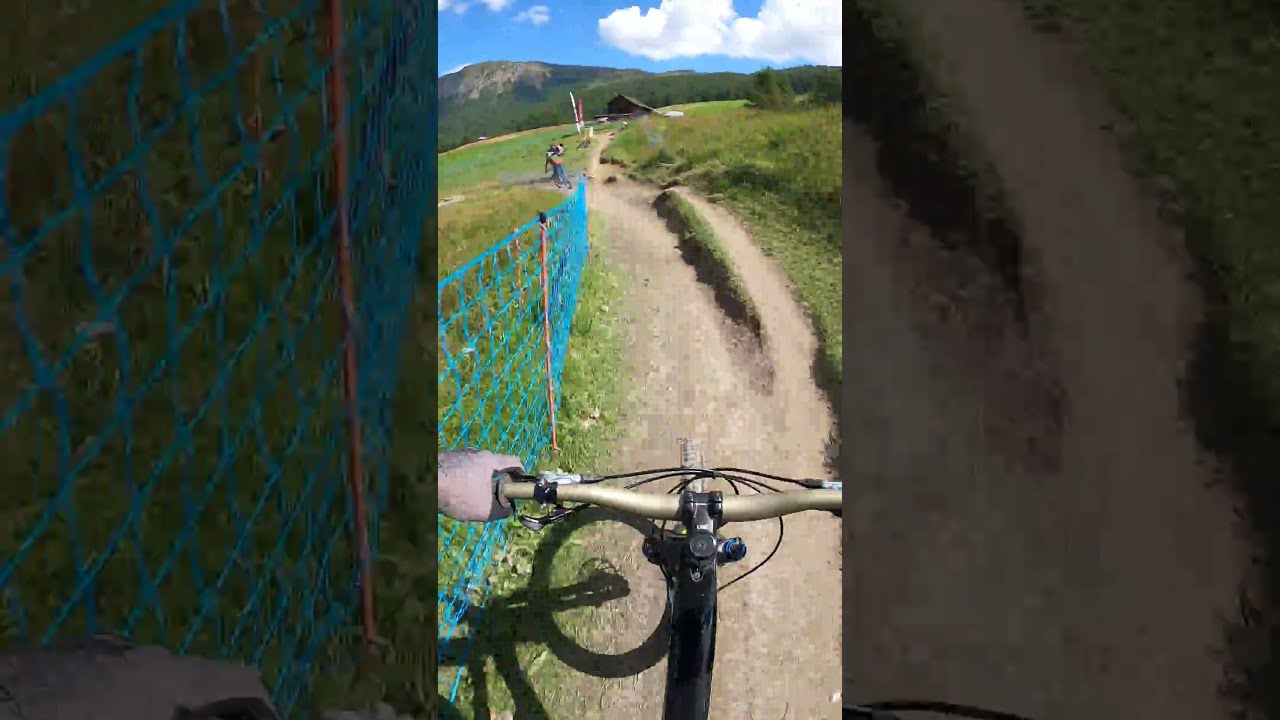The image captures a dynamic scene from a GoPro camera perspective, showing a mountain biker navigating down a light brown dirt trail that cuts through tufts of green grass and scattered weeds. The rider’s left hand, encased in a black glove, grips the gray handlebars tightly, wires from the brake handles leading towards the tires. Shadows of the rider and the bike stretch to the left, partly covering the trail. The trail is dotted with small rocks and reveals slight moisture on the right side. Surrounding the trail, patches of yellowed grass add to the natural landscape.

In the distance, a valley unfolds, hosting a mix of buildings—most notably a red one with a black roof amidst an assortment of indistinguishable structures. Above this townscape, the mountains rise, their peaks shrouded in a misty fog. The scene includes a bright blue sky adorned with clouds, suggesting it is mid-day. The image is divided into three sections: the vibrant central picture and two heavily tinted side sections that zoom in on specific elements—the left focusing on the gloved hand and handlebar, and the right on the moist trail transitioning into the grassy edges.